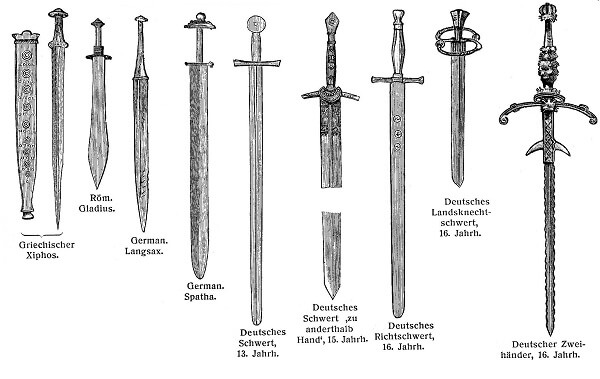In a stark black and white image devoid of borders or background, a meticulous display of various swords and daggers stretches from left to right against the white backdrop of a computer screen. The collection showcases an array of bladed weapons of increasing length, starting with several short swords and extending to longer, more formidable swords. 

On the far right, a double-handed sword with an extensive hand guard stands out due to its impressive size. Next to it, a standard-length sword features a distinctive double-circle hand guard. Following this, a long sword with a simple hilt leads to another hilted weapon, this one distinguished by a leather grip and a pommel.

Continuing the progression, another long sword is notable for its circular hilt and hand guards. Uniquely, the next sword is the only one with a device at the end of the hilt to prevent hand slippage, a functional safety feature. 

Among these, a German sword stands with a long, thin blade and minimalistic handle, lacking a hilt. Further to the left sits a gladius—a shorter sword famous for its wide blade, and finally, a sword of normal length with a scabbard beside it completes the collection. Each weapon’s unique characteristics and the origins or styles they represent are meticulously displayed, offering a comprehensive view of historical and functional sword design.